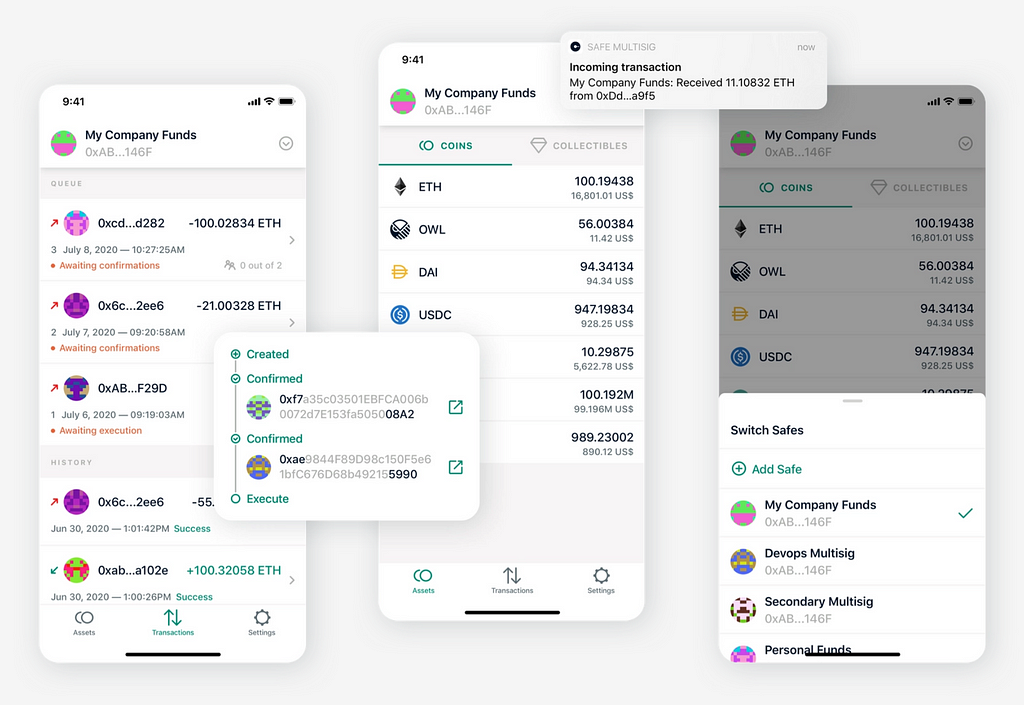In this composite image set against a light gray background, there are three distinct screenshots captured from a cell phone. Let's examine each in detail:

1. **First Screenshot (Left)**:
   - **Background**: White
   - **Top Information**:
     - Time displayed in black text: "9:41"
     - Upper right icons indicating full bars for Wi-Fi and a fully charged battery.
   - **Main Content**:
     - In bold black text: "My Company Funds"
     - To the left, a small cute circle icon that is purple and green.
     - A pull-down arrow on the right side of the text.

2. **Second Screenshot (Middle)**:
   - **Background**: Light gray
   - **Primary Text**: 
     - Displayed prominently: "Q"
     - Below, there is a code: "OXCD D282"
     - Followed by an important value: "-100.02834 ETH"
   - **Bottom Navigation**:
     - Text written in gray: "Assets" on the left, "Transactions" in green in the center, and "Settings" in gray on the right.

3. **Third Screenshot (Right)**:
   - **Visual Flow**:
     - Small green text box reading: "Created", followed by arrows pointing down to "Confirmed", another arrow pointing down to "Confirmed", and finally ending with "Execute".

Each screenshot is a detailed representation of different stages of a digital transaction or summary within a mobile interface, reflecting key financial operations and states, framed by minimalistic and functional design elements typically found in fintech applications.